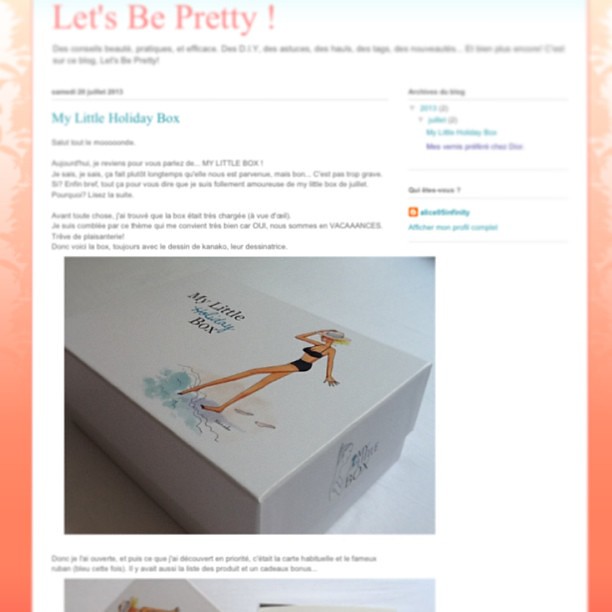The image appears to be a screenshot from a web page featuring a product called "My Little Holiday Box." The central focus is a white box, similar in size to a shoebox, with a prominently displayed picture of a woman in a black bikini and a beach hat, dipping her toes in the water while holding her hat. Above the box, in pink text, it reads "Let's Be Pretty." Below this header, in teal font, it states "My Little Holiday Box." The background of the webpage includes an orange border, and there’s an orange symbol at the top, possibly part of the website's design. The page contains some blurred paragraphs, likely describing the contents of the box, and parts of the text seem to be in French, except for the words "My Little Box." Additionally, there appears to be a dropdown menu to the right and links that suggest further interaction to learn more about the giftable "My Little Holiday Box."